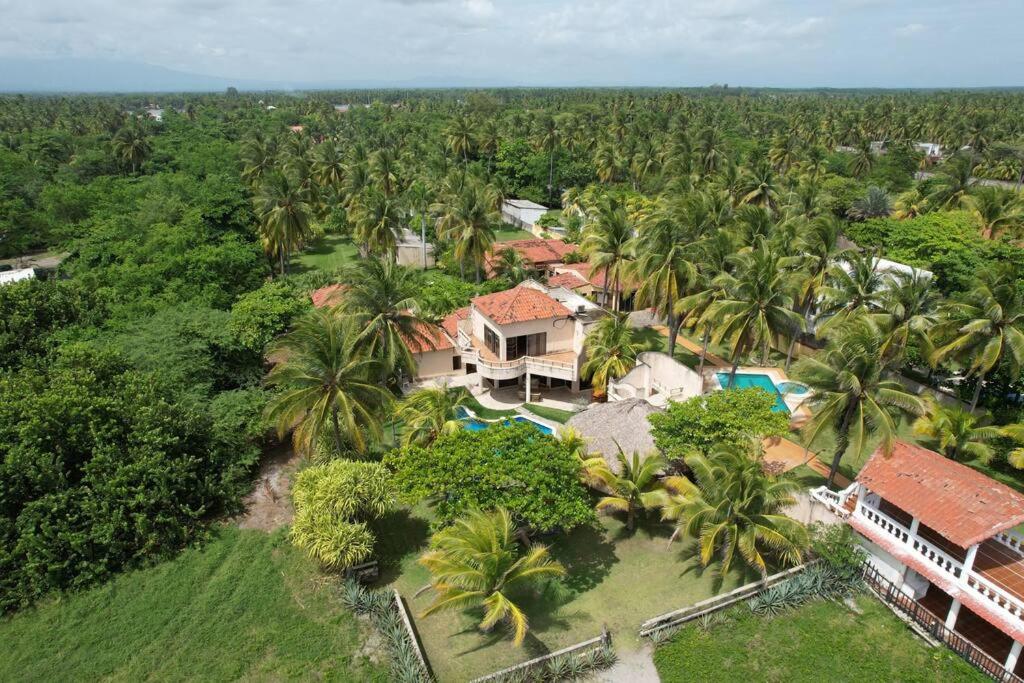The image is a detailed aerial photograph showcasing a lush, tropical estate, likely located in Hawaii. The focal point of the image is a large, high-class residential complex with multiple white-painted buildings featuring terracotta or brick red roofs. At the center is the main building, which has a square structure with a white rail patio or deck. Surrounding the central building are various other structures, including one multi-storied building at the bottom right that has white siding and an open design similar to a pool house.

The estate includes two blue pools, each partially obscured by an abundance of palm trees and other greenery, with one pool situated slightly off to the right and another more centrally located. The property is bordered by fencing and is interspersed with boulders and manicured grassy areas, adding to the lush, green atmosphere. In the background, a dense forest of palm trees and shrubberies envelops the estate, blending into the picturesque landscape. The entire scene suggests an exclusive, possibly communal or resort-like environment, meticulously designed to blend with the tropical surroundings.